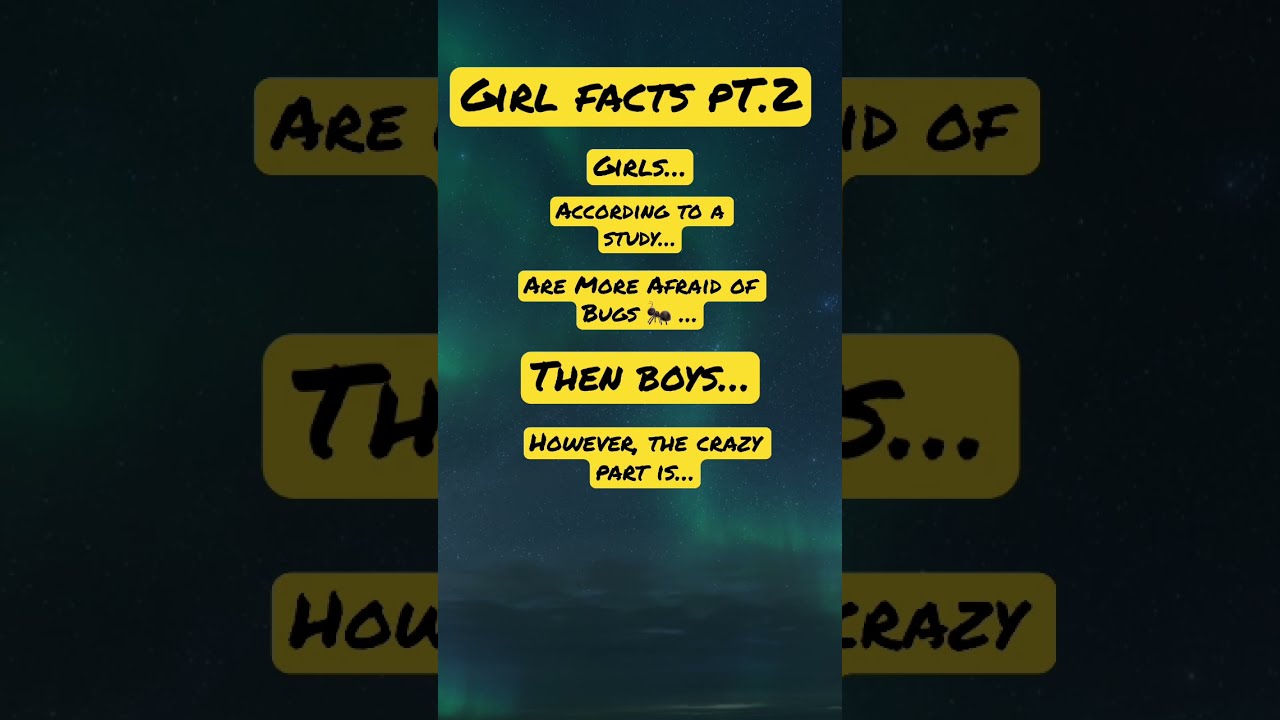The image is a screenshot of a social media video, likely from YouTube Shorts or TikTok, labeled "Girl Facts Part Two" at the top. The background features a nighttime sky with an aurora borealis, displaying greenish lights and stars, adding a surreal, atmospheric touch. The text, written in a playful, marker-like black font, is broken into several incomplete sentences, each underlined by a yellow rectangular overlay that makes it stand out against the backdrop. The fragmented captions read: "Girls... according to a study... are more afraid of bugs 🐜... than boys... however the crazy part is..." but frustratingly, it stops there, leaving the viewer curious about the "crazy part." This interrupted flow of information, combined with the dramatic background, creates a visually striking yet somewhat confusing piece.